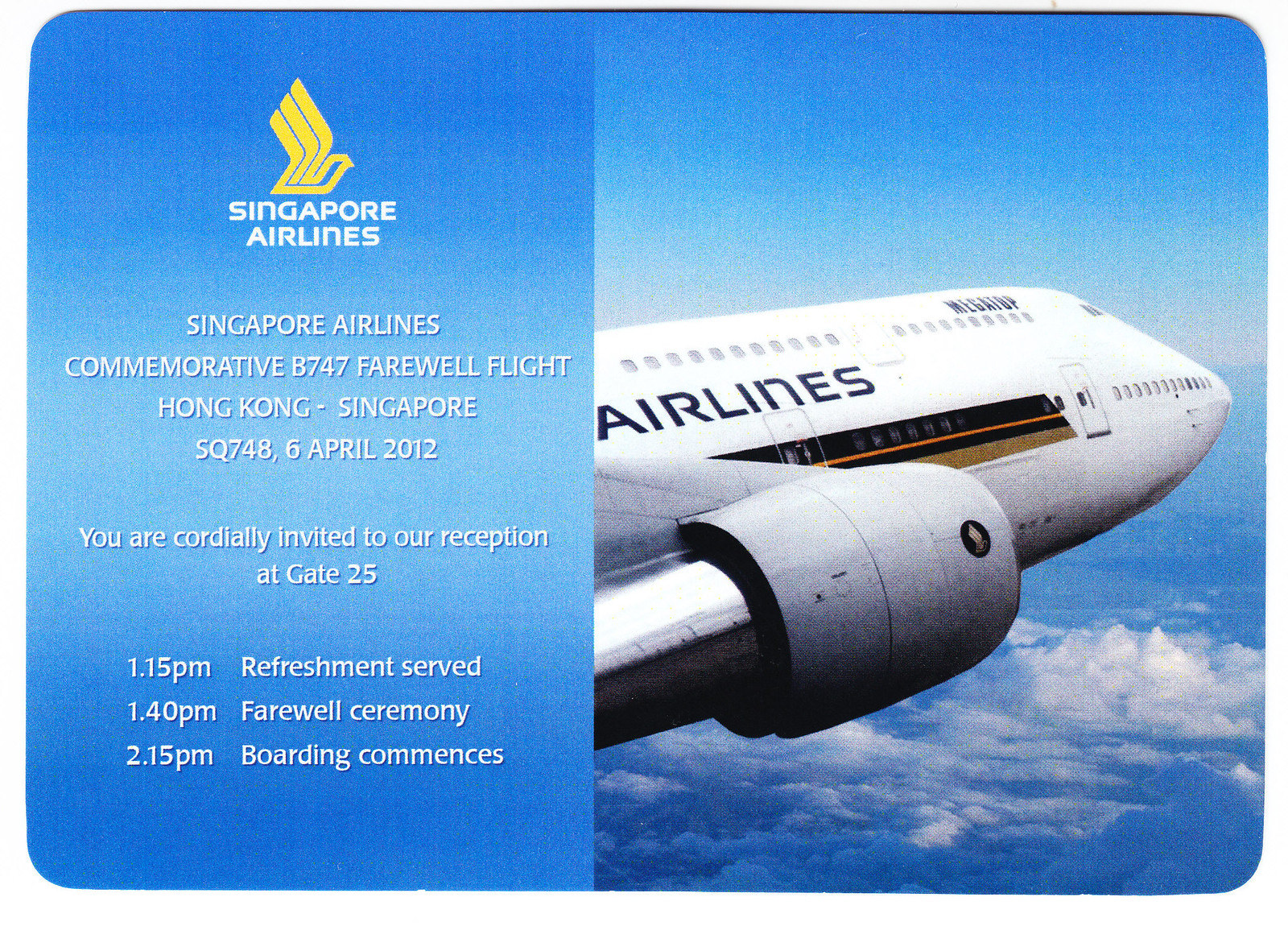This image features an advertising poster divided into two primary sections. On the right, the background showcases a clear blue sky transitioning into white clouds at the bottom. A large, two-story airplane, identified as part of an airline, commands attention in the center. The aircraft is white with two rows of windows, outlined in black, and features a distinct orange, brown, and blue stripe running along its length. The visible front part displays the cockpit, engines, and the word "Airlines" prominently written on the fuselage. 

On the left side, set against a predominantly blue background, there is a yellow bird logo at the top, accompanied by the heading "Singapore Airlines" in white letters. Below it is detailed text that reads: "Singapore Airlines Commemorative B747 Farewell Flight, Hong Kong to Singapore, SQ748, 6 April 2012. You are cordially invited to our reception at Gate 25. 1:15 PM, Refreshments served. 1:40 PM, Farewell ceremony. 2:15 PM, Boarding commences."

The poster seems to be digitally generated and serves as an invitation to a special farewell flight event, providing detailed information about the ceremony and flight schedule.